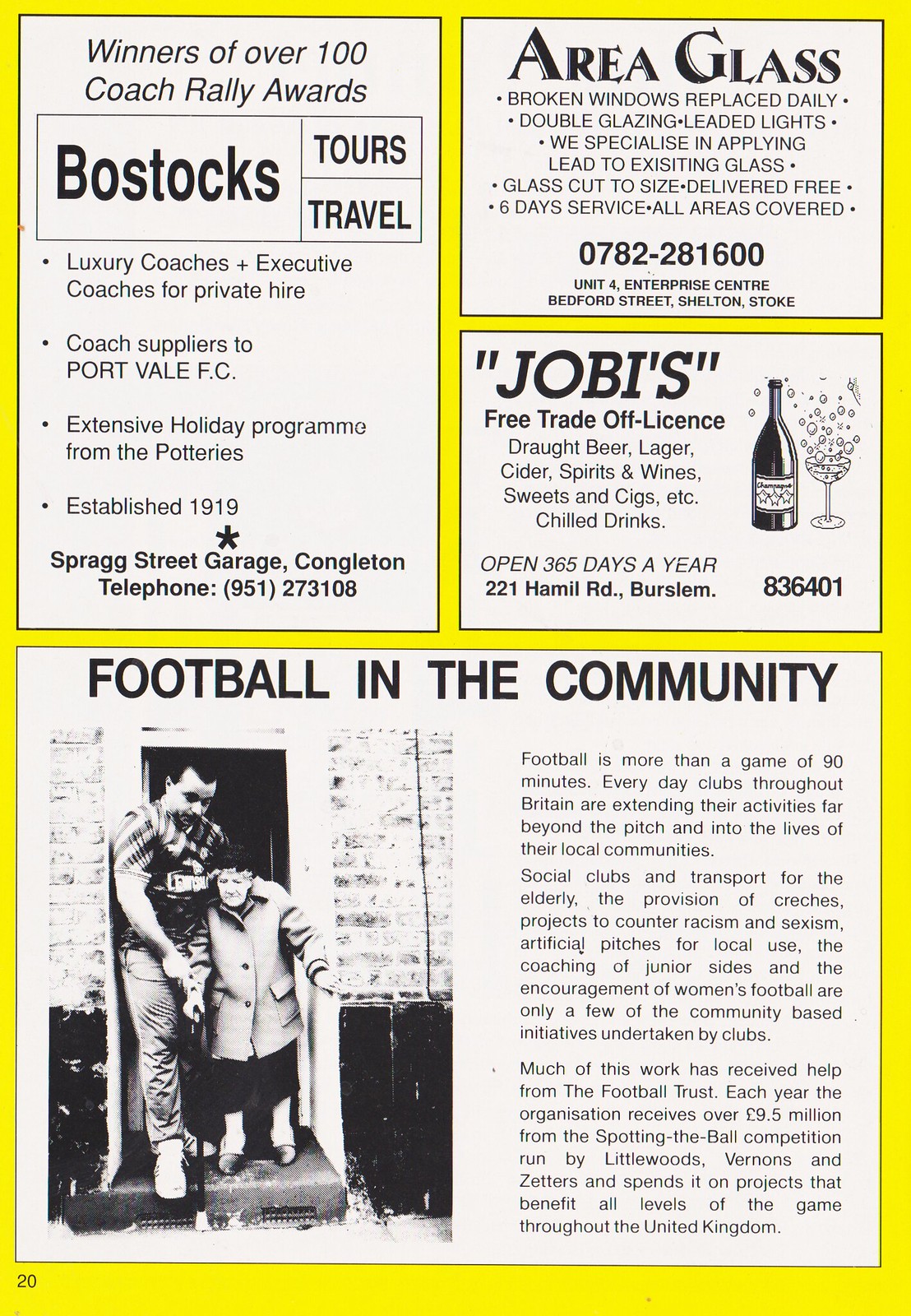This page from an old European football magazine features a yellow background with four distinct advertisements, each set in white boxes with black text. The top-left box promotes Bostock's Tours and Travel, winners of over a hundred coach rally awards, offering luxury and executive coaches for private hire, alongside additional service details. To the right, the top box advertises Area Glass, specializing in replacing broken windows daily, applying leaded lights, double glazing, and providing a contact phone number. Below that, an ad for Jobi's Free Trade Off-License highlights their offerings of beer, lager, cider, spirits, wine, sweets, and chilled drinks, with the inclusion of an address. Dominating the bottom half of the page is an article titled "Football in the Community," featuring a black-and-white image of a tall, muscular football player assisting a frail elderly woman out of a brick building. The article details the community involvement initiatives connected to football.